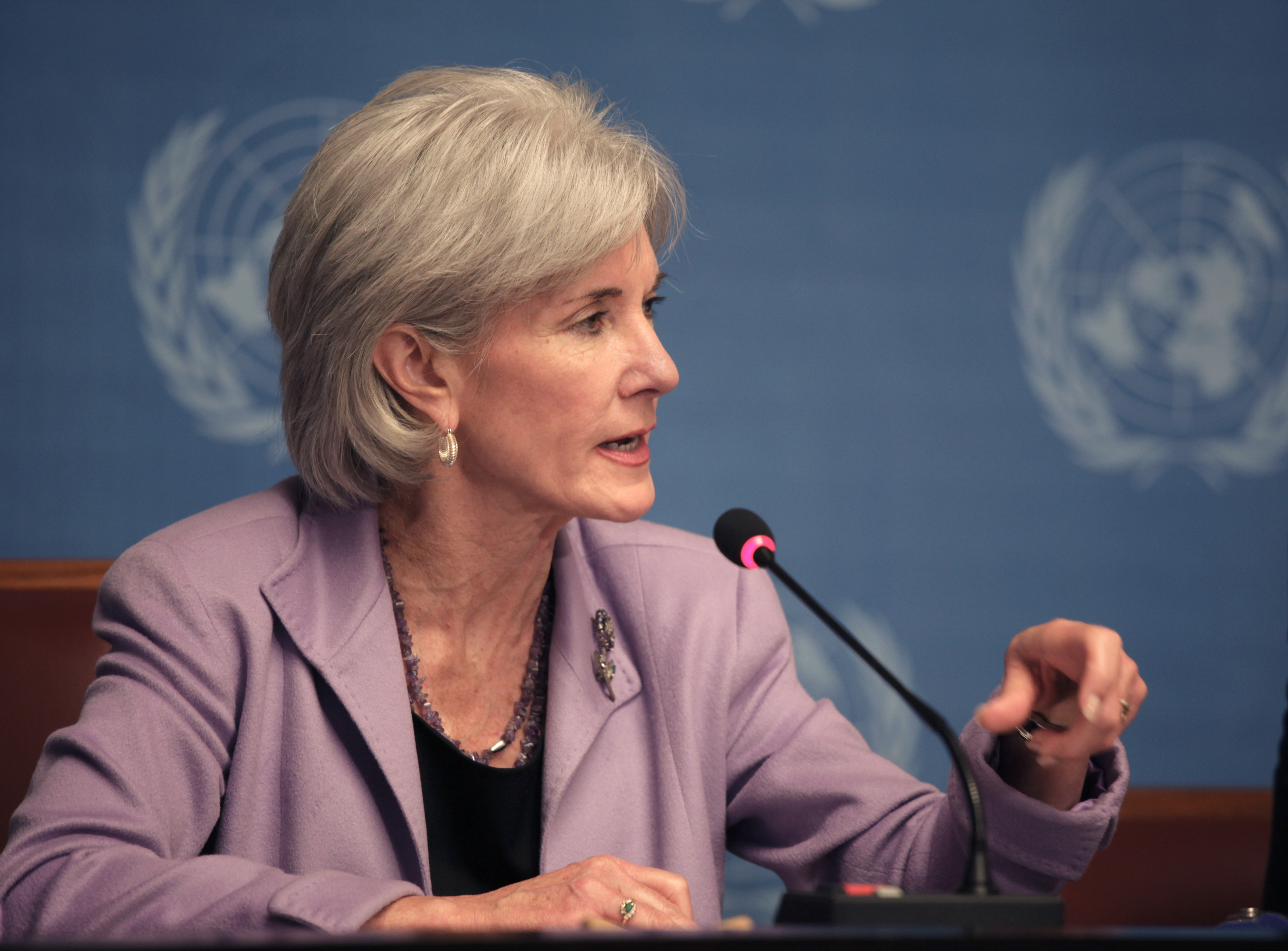In this detailed image, a seated white female, likely of the United Nations, is seen speaking into a microphone while gesturing with her left hand. She is attired in a lavender business jacket with a noticeable pin attached to the left collar, complemented by a black shirt underneath. Her attire includes a double-strand grayish-purple necklace, a brooch, and rings on her fingers, indicating diamond and gold details. The woman, with short blonde hair neatly tucked behind her ear, has a stern expression and slightly open mouth, revealing the bottom row of her teeth as she speaks and points. She also sports dangling silver or gold earrings. The background prominently features a blue backdrop with the white UN logo, characterized by an image of the world surrounded by leaf-like decorations. The scene includes elements of brown wood in front and behind her, and the microphone, adorned with a pink area beneath it, is mounted on a box with yellow and white buttons.